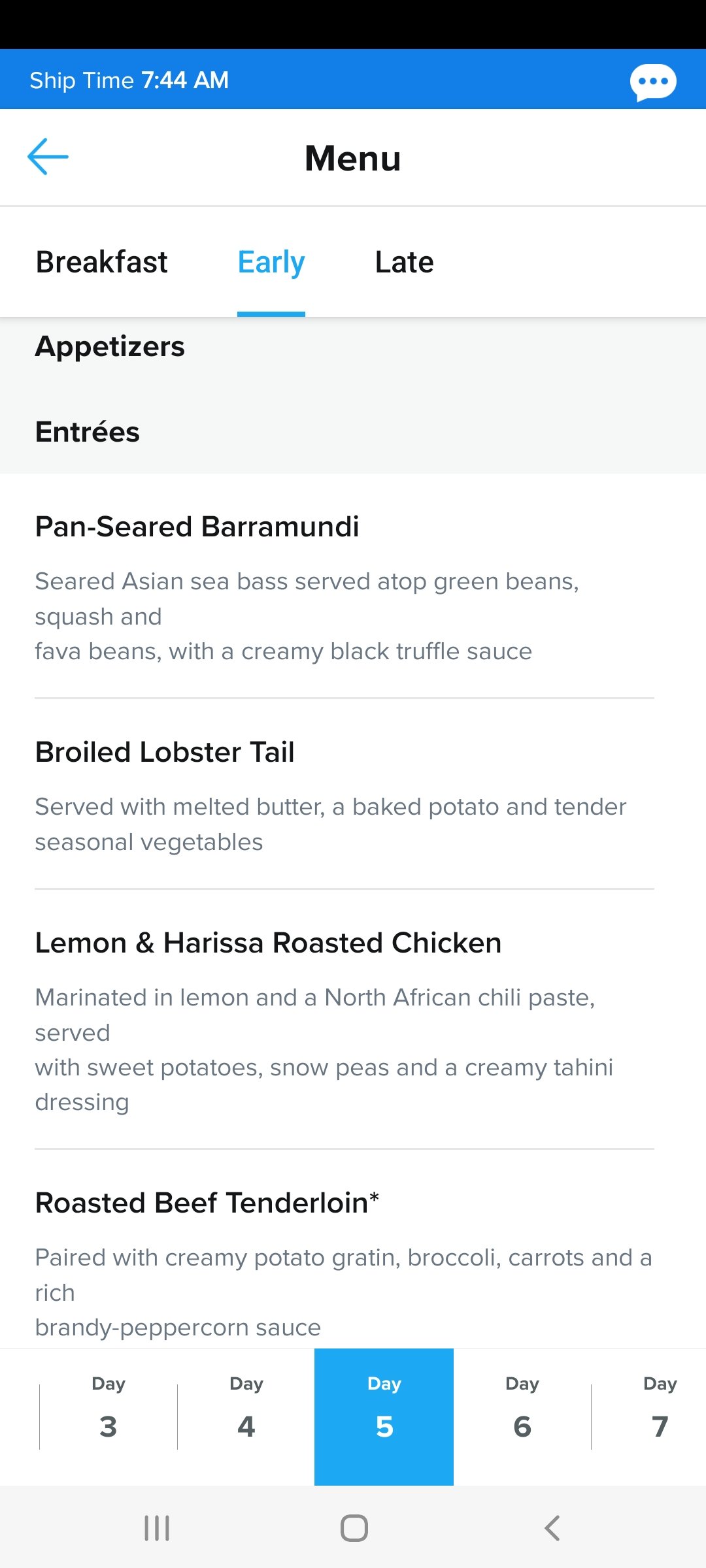This image, captured from a smartphone, features a detailed view of a menu page. At the top of the screen, a black banner spans the entire width of the phone. Directly below, a blue banner with white, bold text reads "Ship Time: 7:44 AM." To the right, a white, speech-bubble icon with three dots is visible.

Beneath these banners, the word "Menu" appears in bold black text, accompanied by a left-facing arrow on its left side, indicating the option to go back. The menu is divided into sections starting with "Breakfast," followed by "Early" and "Late." "Early" is highlighted in blue and underlined, indicating that this page is dedicated to the early menu.

The early menu lists its items starting with a light gray box titled "Appetizers" in bold black letters. Below it, the "Entrees" section begins with the first item: "Pan-Seared Barramundi," highlighted in bold black lettering. The description below it, in gray text, reads, "Seared Asian sea bass served atop green beans, squash, and fava beans with a creamy black truffle sauce."

Other entrees include:

- "Broiled Lobster Tail" with its description.
- "Lemon and Harissa Roasted Chicken" with a description.
- "Roasted Beef Tenderloin," also detailed with a description.

Towards the bottom of the menu, days 3 through 7 are listed in black text, with "Day 5" highlighted in blue. Below these, there are additional navigation options featuring icons: three horizontal lines, a small square, and a back arrow.

This comprehensive caption provides a vivid and structured description of the menu page displayed on the smartphone screen.